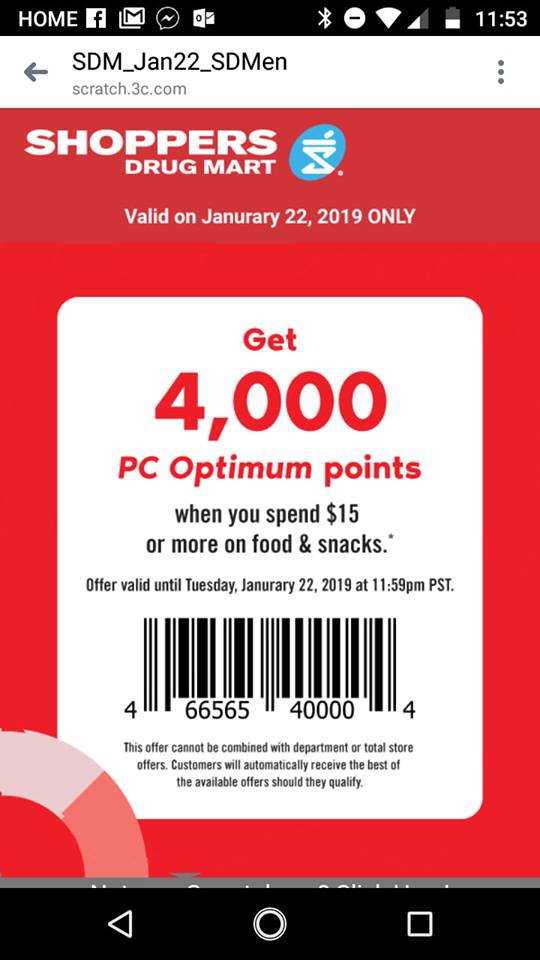The screenshot depicts a cell phone screen showcasing a promotional offer. 

At the very top, a narrow black bar spans horizontally, occupying roughly the top 5% of the screen. Within this bar, white icons and text include "Home" on the far left, followed by a Facebook icon, a Gmail icon, a chat bubble, and a mail icon. On the far right of the bar, two signal strength indicators, a half-filled battery icon, and the time "11:53" are displayed.

Immediately below, a wider white bar follows, containing a gray left arrow and a title reading "SDM_Jan 22_SD men." Below the title, in small gray text, is the URL "scratch.3c.com." On the right-hand side of this bar are three vertical dots.

The dominant portion of the screen features a red background with large white letters in the center reading "Shoppers," followed by smaller text "Drug Mart." This branding is accompanied by an icon on the right that is light blue and oval-shaped, tilted towards the 1 o'clock position. The icon contains a horizontal white line with a backward "Z" shape beneath it.

At the bottom of the screen, it states, "Valid on January 22, 2019, only." Further down, a promotional message reads, "Get 4,000 PC Optimum points when you spend $15 or more on food and snacks."